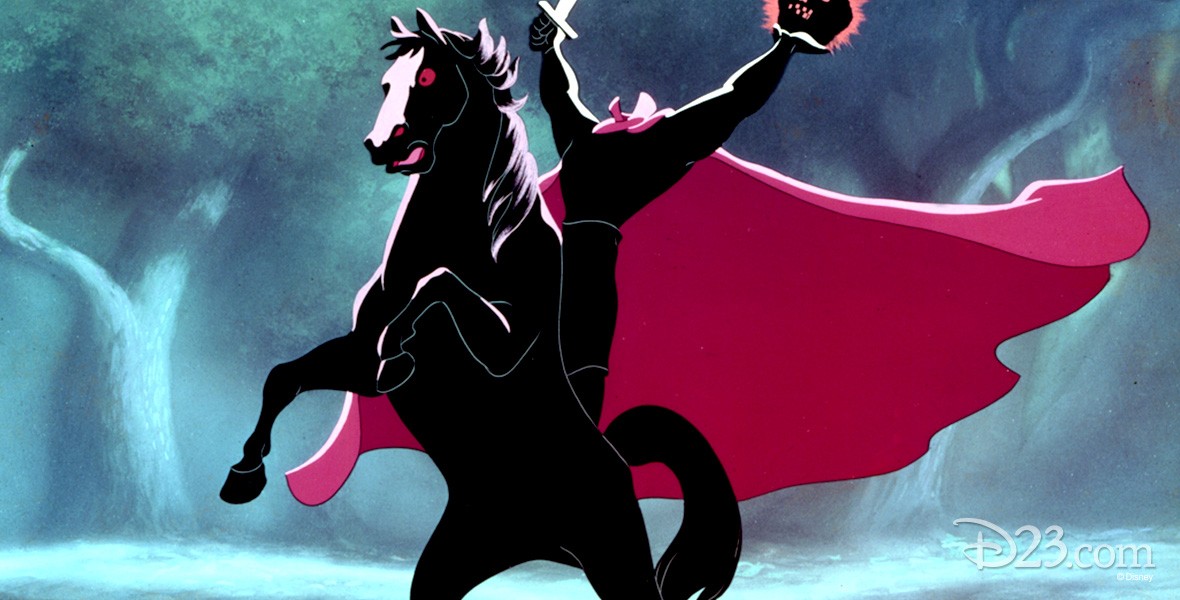This detailed image captures a vivid still frame from a classic Disney cartoon, believed to be "The Legend of Sleepy Hollow." Central to the composition is the iconic Headless Horseman, dramatically positioned astride a black horse rearing on its hind legs. The horse is striking, with ominous red eyes, nostrils, and mouth, and its mane and forehead are highlighted white, likely by moonlight. The Horseman is equally formidable, clad entirely in black, distinguished by a flowing red cape with a prominent red collar. In his right hand, he brandishes a sword, while his left hand raises his glowing, severed head, which resembles a fiery jack-o-lantern. The background features a soft, old-school painted forest, evoking a haunting nighttime ambiance. Adding authenticity, a Disney watermark, "D23.com," is visible in the bottom right corner. The wide array of colors—burgundy, pinkish red, black, red, pink, greens, blues, whites—enhances the eerie yet mesmerizing scene, making it a quintessential depiction of the Headless Horseman from Disney lore.